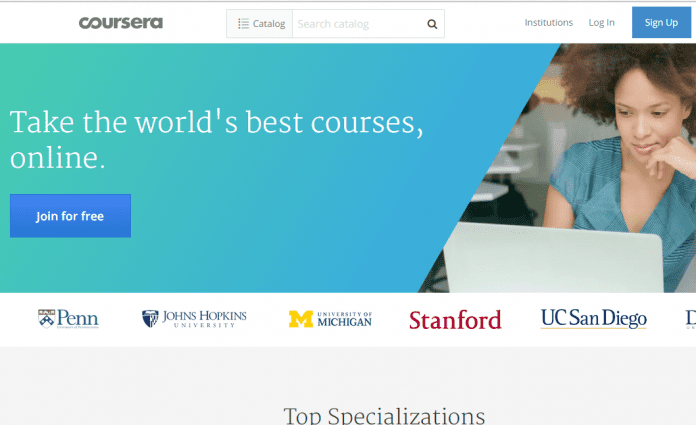Coursera Promotional Visual: 

The Coursera homepage features a clean, teal-themed design. Dominating the visual is an African-American woman with beautiful, natural hair, clad in a matching teal blouse. She is seated in front of a laptop, symbolizing the platform's online learning environment. 

In the foreground, a prominent blue button encourages users to "Join for Free," highlighting the accessibility of the platform. Coursera, a renowned online learning hub, offers courses from esteemed institutions such as Penn State, Johns Hopkins University, University of Michigan, Stanford, and UC San Diego. 

Though the image itself doesn't list these specializations, the interface suggests easy navigation to explore various courses via a search menu. The headline "Take the world's best courses online" underscores Coursera's mission to provide top-tier education that can enhance job prospects, professional skills, or personal development. 

This visual serves as the login screen, inviting users to embark on an enriching educational journey.